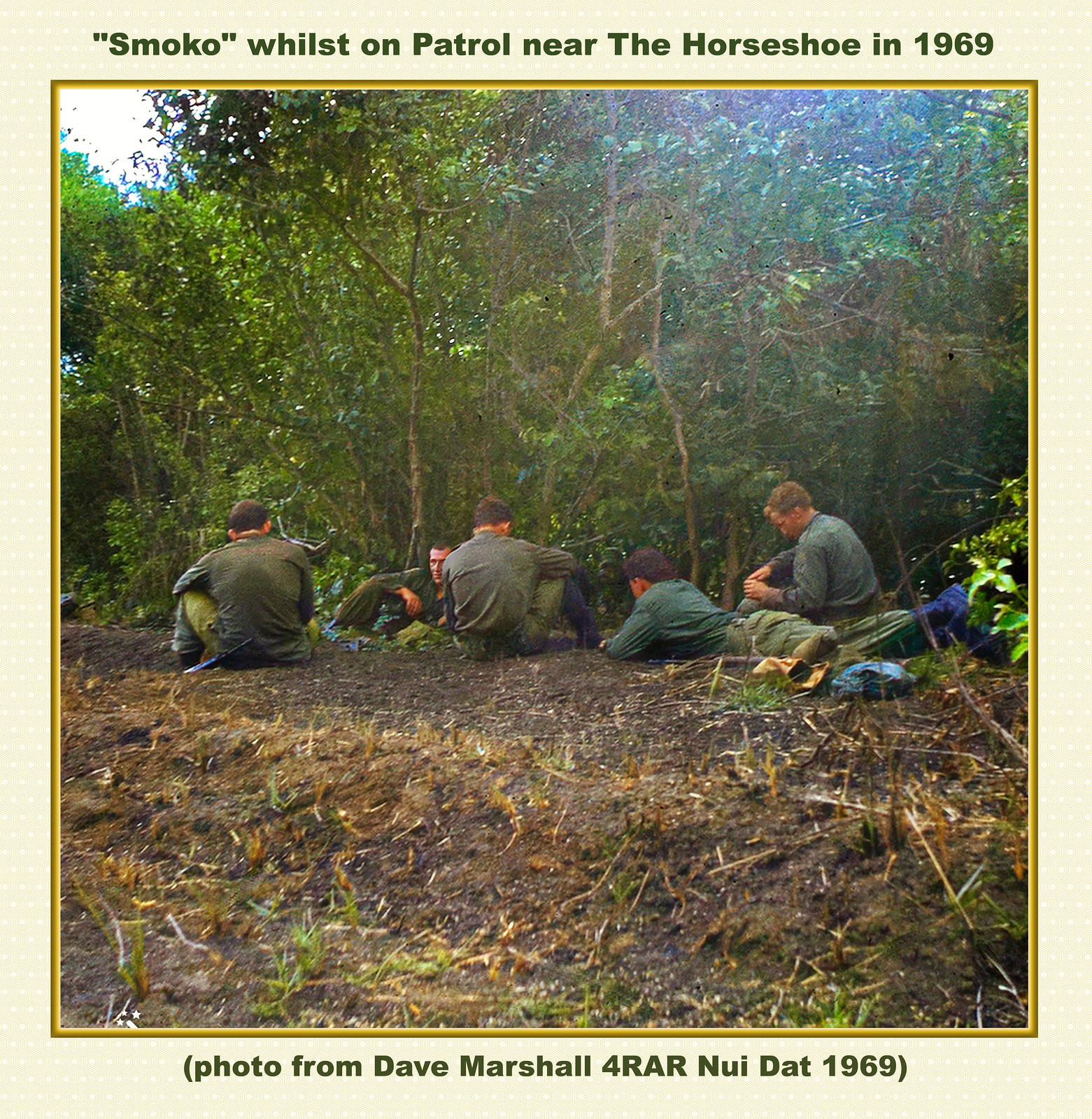This is a color photograph, framed with a yellow border, taken during the Vietnam War in 1969. The caption at the top reads, "Smoko, whilst on patrol near the Horseshoe in 1969," and the bottom attribution states, "Photo from Dave Marshall for RAR Nui Dat 1969." The image features five men in green fatigues, either sitting or lying on the ground in a vegetated area. Four men sit with their backs mostly turned to the camera, while one man lies on his stomach and another man’s side profile is visible. The ground they occupy is a mix of dark brown dirt with sparse vegetation, including some brown and green stalks. The background reveals a dense cluster of white-barked trees, which appear almost like vines in places, indicative of a thick, bushy environment.